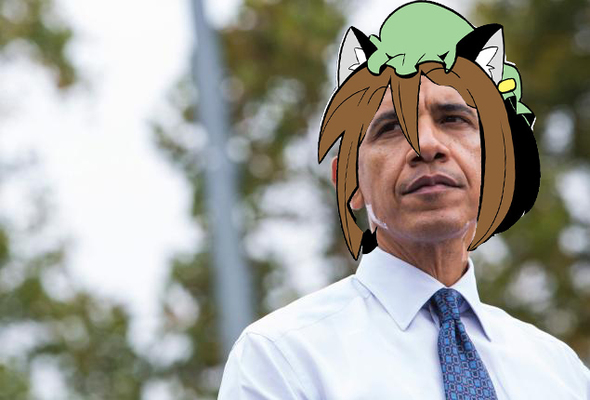In this humorous, edited photograph of President Barack Obama, he is seen wearing a white button-up collared shirt paired with a blue textured tie, typical of his professional attire. However, the image has been playfully altered with a superimposed cartoon headdress featuring a character with brown hair in the front and black hair in the back. The character’s headdress includes black and white cat-like ears and a green bonnet. The background is blurred, showing a daytime outdoor setting with indistinct metal posts, possibly flagpoles, and lush green tree branches, suggesting it might be overcast. Despite the playful additions, Obama’s composed expression contrasts with the whimsical cartoon elements added to the photo.